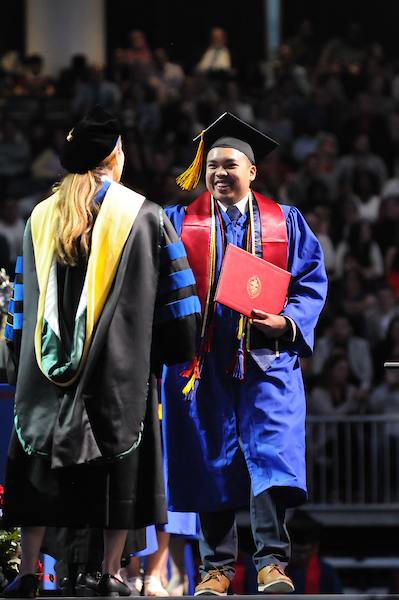The photograph captures a significant moment during a graduation ceremony, with a focus on two central figures on stage amidst a large crowd seated behind a metal gate in the background. The woman, on the left, is facing away from the camera, her golden hair tied in a ponytail and adorned with a black graduation cap and gown, paired with black shoes. Opposite her, to the right, stands a smiling man dressed in a blue jacket and red shawl with a black graduation hat trimmed in yellow. His right hand holds a red diploma featuring a subtle gold insignia and his brown shoes complete the ensemble. The scene is lively with varied colors including black, yellow, green, tan, red, white, brown, and gray, set in an indoor venue with no visible text. The crowd, though blurred, is a sea of anticipation and support, enhancing the celebratory atmosphere.